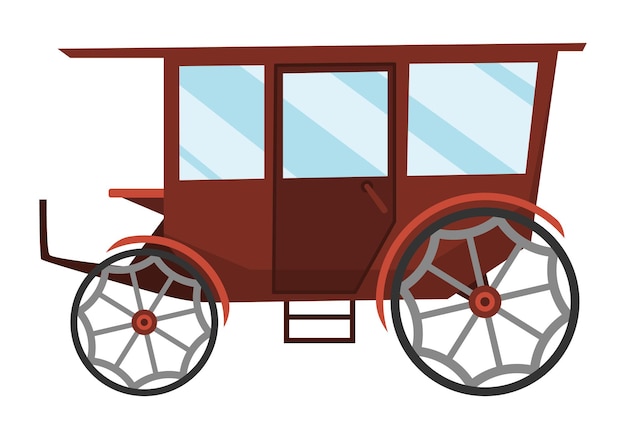The image features a hand-drawn, cartoon-style horse-drawn carriage set against a solid white background. The carriage is predominantly burgundy-red, with a darker shade for the central door. It has three large, diagonally-striped blue windows and a set of small black footstools beneath the door for easy access. The roof extends slightly over the front, where a small seat is positioned for the carriage driver, along with a mounting point for attaching horses. The two wheels, distinguished by their thin black tires and hexagonal-spoked rims with burgundy-red center caps, vary slightly in size, with the back wheel being larger than the front. The image's simplistic features are accentuated by the blank white background, emphasizing the carriage's detailed artistic elements.